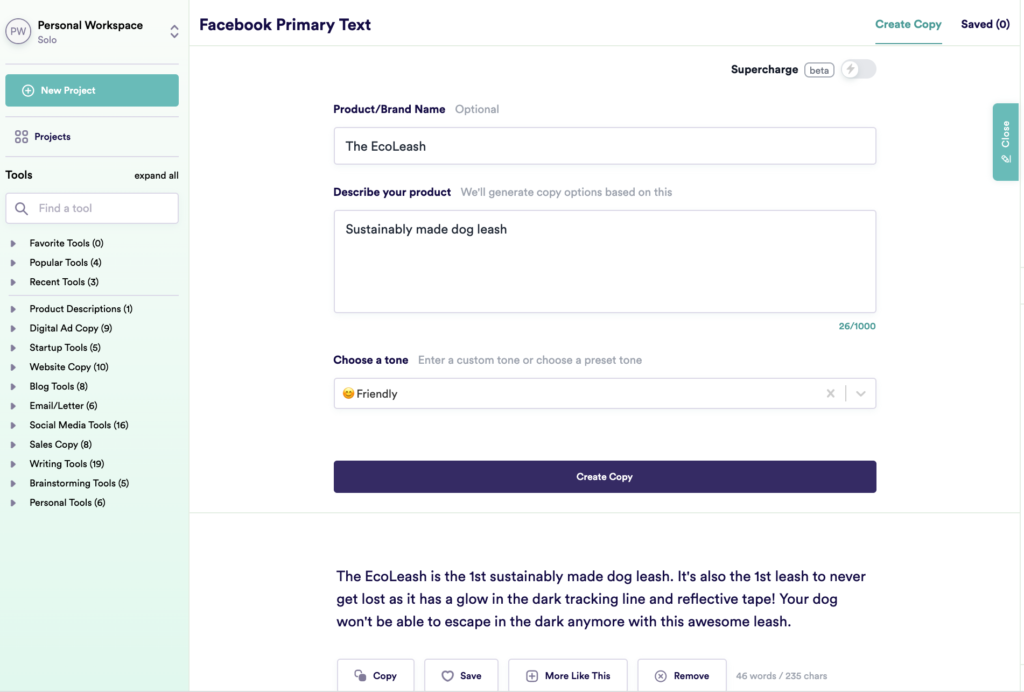This image is a screenshot of a web page featuring a user interface for a personal workspace. The left sidebar has a gradient background that transitions from mint green at the bottom to nearly white at the top. At the top left corner of the sidebar, there is a light grey circle with a dark grey outline. Inside the circle, dark grey text reads "PW." To the right, black text reads "Personal Workspace," and below this, justified to the left, light grey text reads "Solo." To the right of this text, there are two arrows: one pointing up and one pointing down. Beneath this section, a thin line separates it from a teal button labeled "New Project," which features a white plus icon to the right of the text. Another thin line separates this button from the next section, which starts with bold text reading "Projects" next to an icon of four squares arranged in a 2x2 grid. 

Underneath this section is another thin line, followed by a section titled "Tools" in black text at the top left and "Expand All" in smaller text at the top right. Below this, there is a search bar displaying light grey placeholder text, "Find a Tool," accompanied by a light grey magnifying glass icon to its left. A list of tools, represented by lines of black text, appears below the search bar.

The main body of the webpage has a white background. In the top left, bluish-grey text reads "Facebook Primary Text." At the top right, there are two options: one is "Create Copy" in teal with a teal underline, and to its right, "Saved (0)" in bluish-grey text. Underneath this header, a thin line aligns with the teal underline. Lower on the right side, the black text "Supercharge" is followed by grey text reading "beta" with a grey outline around it. To the right of this, there is a selection button featuring a white circle on the left with a light grey lightning bolt icon inside, enclosed within a light grey pill shape. Below this, there are additional text entry boxes, titles, and lines of text.